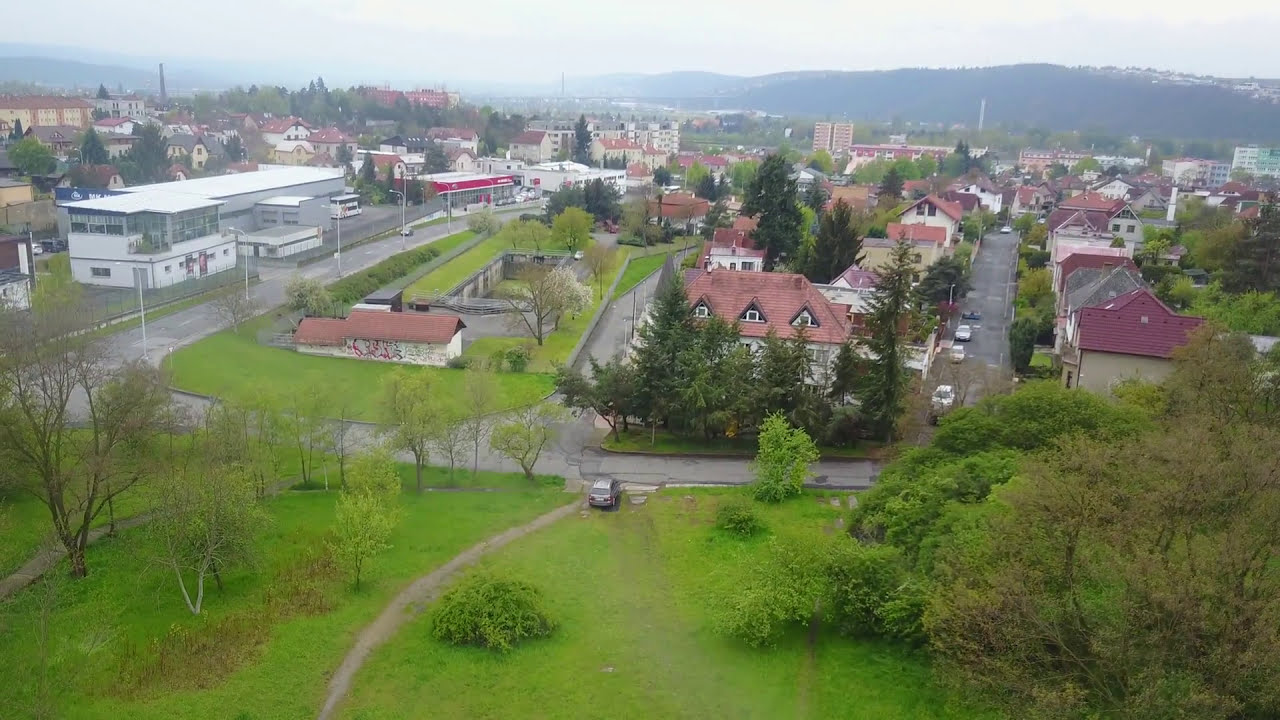This high-resolution daytime aerial photograph captures an idyllic European residential town, showcasing its meticulously planned architecture and lush green spaces. The image is captured in landscape orientation, revealing a panoramic view from an elevated position, likely from a drone or airplane.

In the center right of the image, numerous two- and three-story Tudor-style homes with red and light gray roofs line straight, tree-adorned streets. These houses are nestled among beautifully maintained lawns and gardens, creating a picturesque community atmosphere. Scattered throughout the residential areas are several cars, either parked or driving along the streets.

On the left-hand side of the photo, distinguishing itself from the residential sector, is a larger, paved highway running vertically from the mid-horizontal section to the upper center left. Adjacent to this highway stands a prominent two-story white building, possibly a transit station or hub, with a flat roof and what appears to be a large vehicle in its center.

In the lower third of the image sits a verdant park, marked by a narrow paved path that meanders from left to right. The park exhibits diverse natural features, such as dense trees in the lower right corner, a small grove in the lower left corner, and a field of manicured grass in the center. The foliage hints at the transition to fall, suggesting the photo was taken in late summer or early autumn.

Beyond the town, the upper third of the image is dominated by a smooth, flat mountain range stretching horizontally. This elevated landmass is dotted with additional buildings, leading up to a misty mountain and the horizon where a cloudy grayish-blue sky looms.

Additionally, a few commercial structures are visible, including a one-floor building with a red awning and large windows on the left-hand side, as well as a notable tower in the top left of the image. Moreover, a sunken courtyard or possible grass-roofed structure can be seen in the center, enhancing the town’s architectural diversity.

Overall, this detailed photograph splendidly captures the serene yet structured essence of a European town nestled against a picturesque mountainous backdrop under a muted, overcast sky.